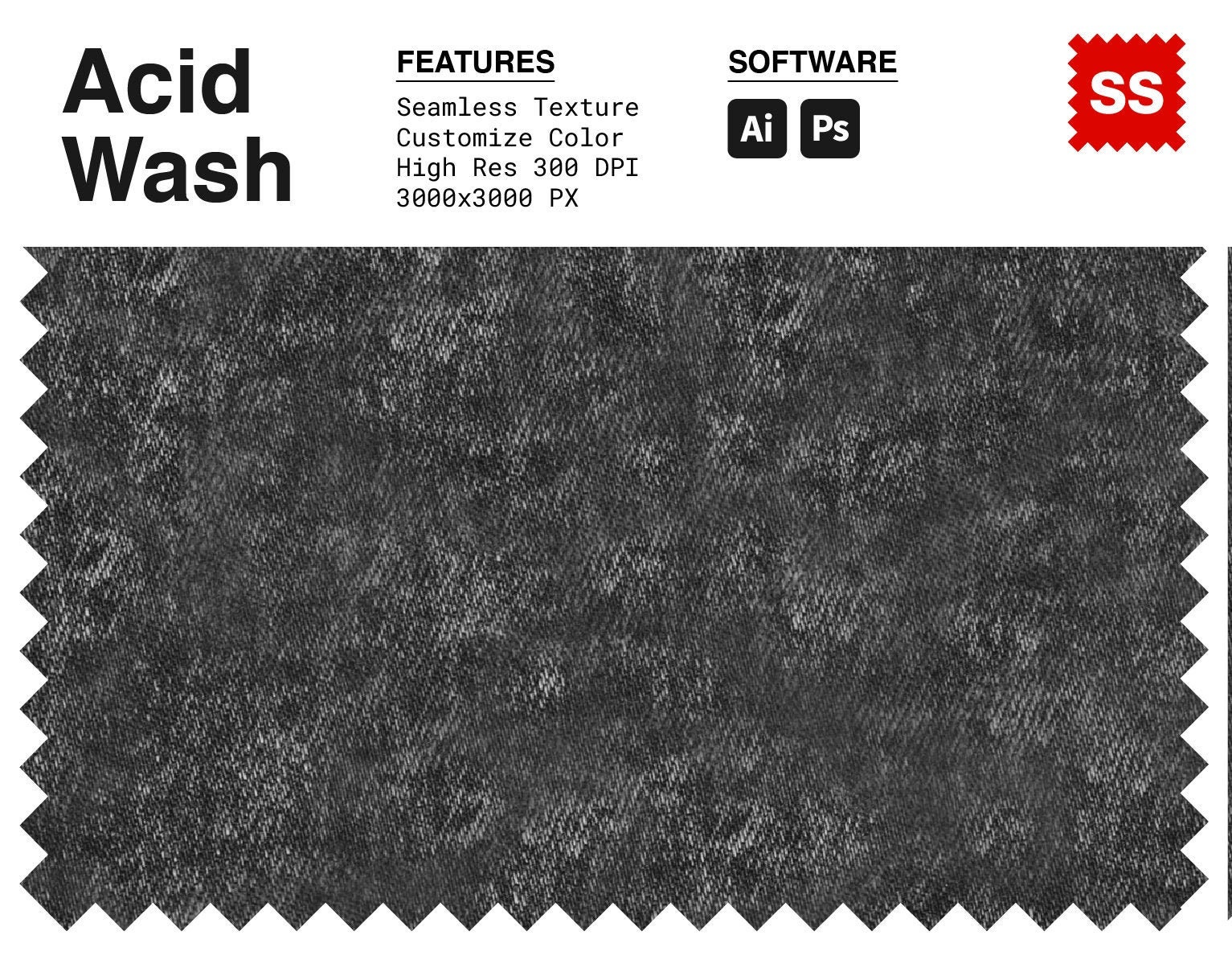The image depicts a swatch of acid-wash denim fabric with a zigzag cut on three sides, positioned on a white background. The top edge of the fabric is smooth, and a narrow black line runs down the right side. At the top left, bold black text reads "Acid Wash." Directly to the right, block letters underline the word "Features," followed by a list in smaller black text: "Seamless Texture," "Customized Color," "High Resolution 300 DPI," and "3000 x 3000 PX." Next to these features, the words "Software AI" and "PS" are presented in black boxes, indicating compatibility with AI (Adobe Illustrator) and PS (Photoshop). On the far right, a red square with a zigzag border contains two white "S" letters. This composition serves as an advertisement for acid-wash denim, highlighting its features and the software tools used for its creation.